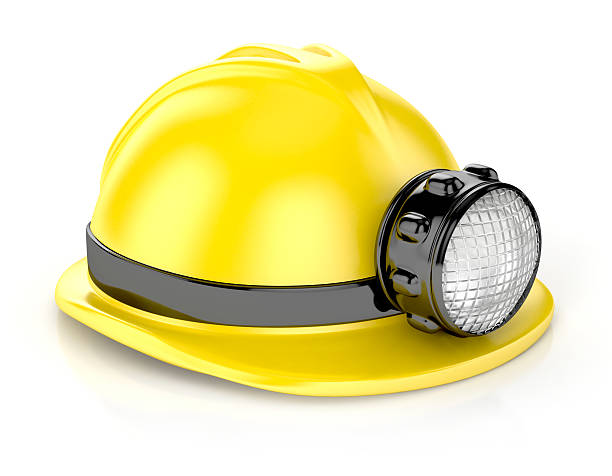This close-up image features a bright yellow hard hat, notable for its compact size which suggests it might be suitable for a child or be a specialized model. The hard hat has three raised ridges at the top, converging in the center to provide extra structural protection. A solid yellow brim extends uniformly around the edge of the hat. 

Encircling the hat is a shiny black band, adding a contrasting accent to the bright yellow surface. Prominently attached to the front of this black band is a round light, enclosed in a black plastic frame adorned with small uniform knobs likely for grip and easy operation. The bright white light is shielded by a glass lens, featuring a grid pattern of evenly spaced squares, further enhancing its utility in dark environments such as mining.